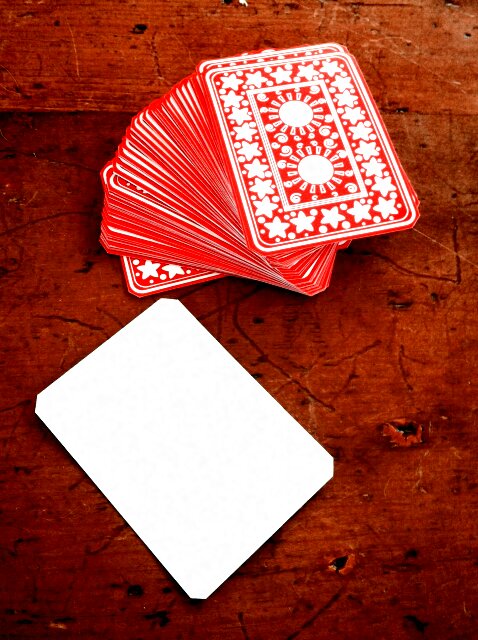The image portrays an old, worn wooden table or crate, characterized by visible knots and numerous scratches, reflecting its aged condition. On this rustic surface, a deck of cards is artfully splayed out. The cards feature red backgrounds with intricate white designs. The outer rims of the cards are adorned with white stars, and within the inner rectangle of each card, two white suns are prominently displayed. The geometric design of the white stars and suns hints at an oriental-inspired motif. At the bottom of the image, one card stands out, flipped over, displaying a completely blank white face, isolated from the spread of the other detailed cards above.